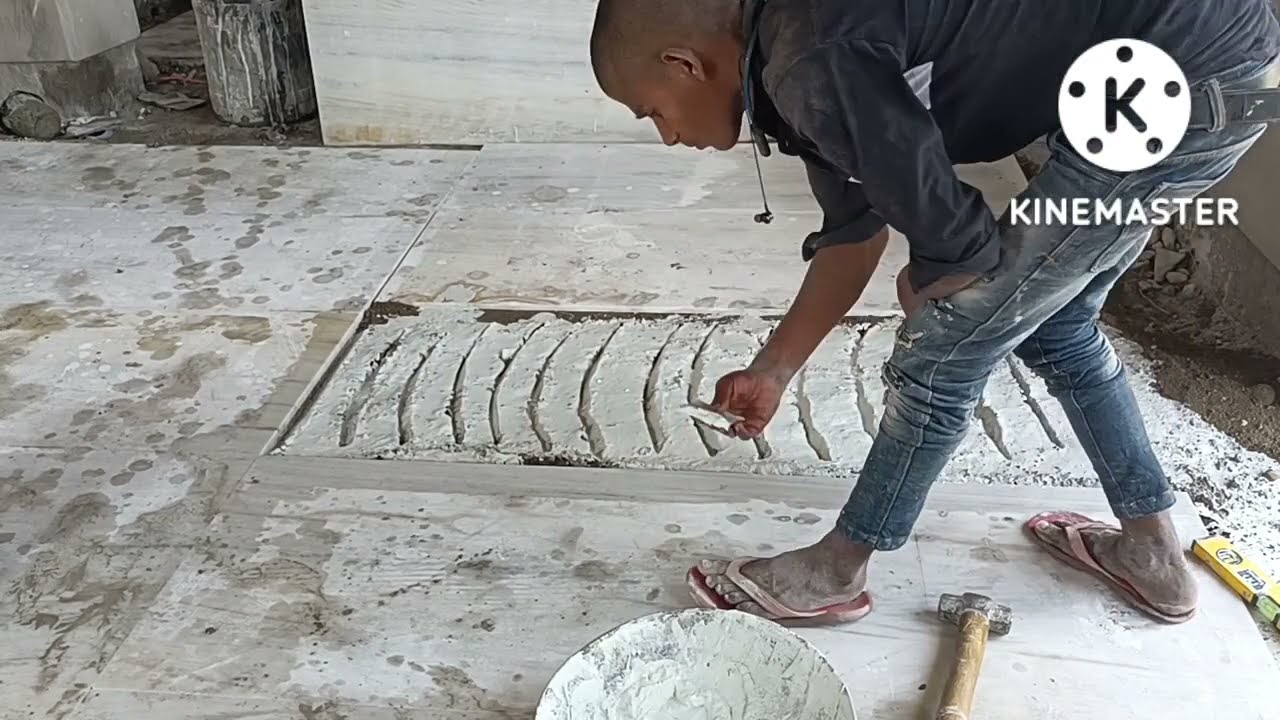In the image, a young man with brown skin and a bald head, wearing a long-sleeved blue hoodie and skinny blue jeans, is working on a large concrete platform that seems to be under repair. He is barefoot, with his feet coated in white concrete powder, suggestive of an arduous day at work, and he is wearing flip-flops which are placed aside. The man is bent forward, one hand on his knee and the other holding a concrete trowel, smoothing fresh concrete within a cut-out rectangular section of the platform. Around his feet lie various tools, including a small hand-held sledgehammer and a level. A bowl with concrete mixture is positioned near his left foot, underscoring the active construction environment. To the right side of the image, there is a circular white logo resembling an artist's palette with five holes and a cutout 'K' in the center, underlined by the word 'KINDMASTER' in white capital block letters. The background reveals a gravel surface bordered with some white paint and other equipment like a bucket, further highlighting the ongoing construction work.